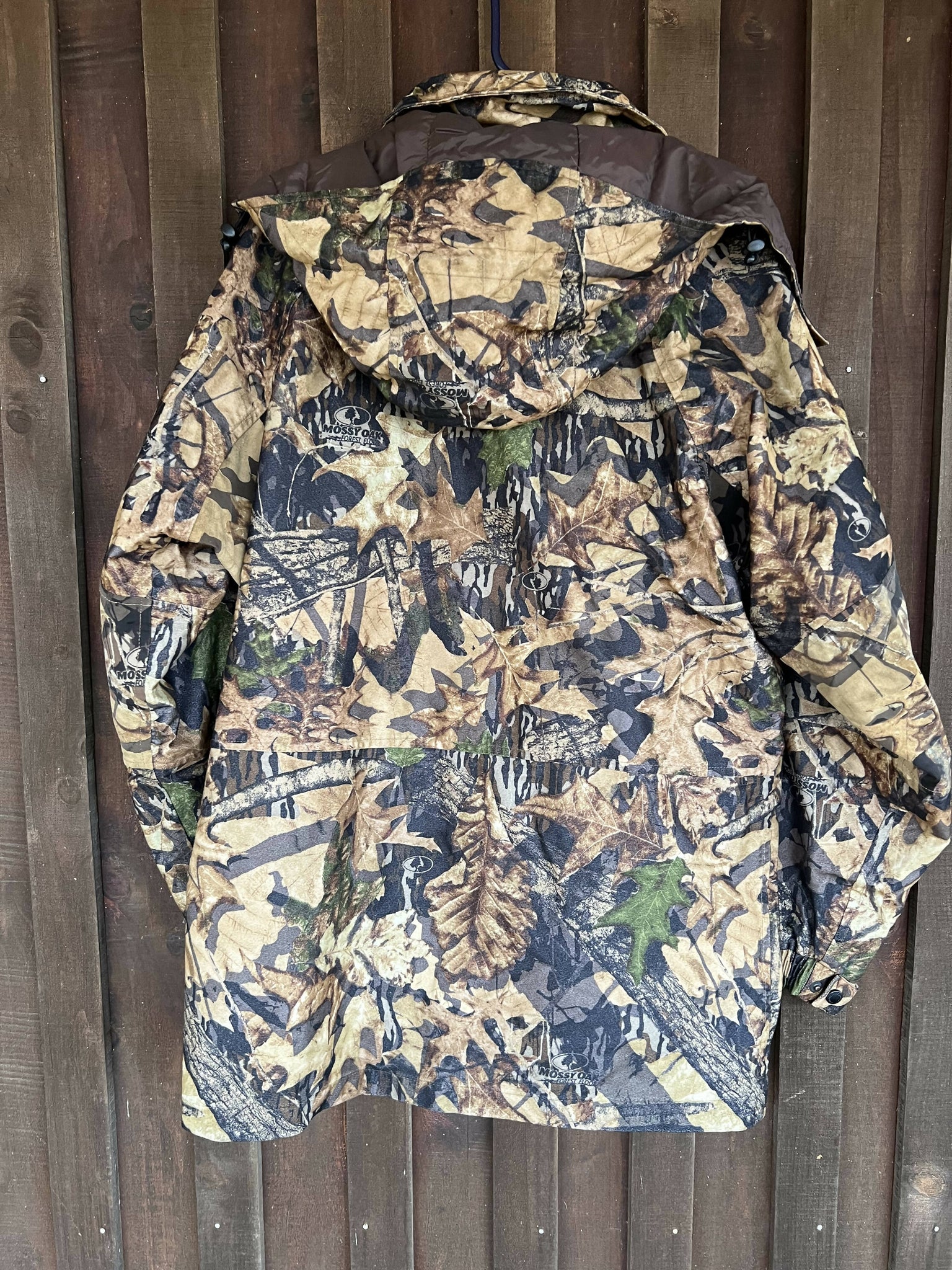The image features a detailed camouflage hunter’s jacket, prominently displayed on a black plastic hanger against a rugged wooden wall, possibly the side of a shed. The wood, characterized by its dark brown and grayish tones, is accentuated with silver nails. Viewed from the back, the jacket showcases an all-over print of leaves, branches, and trees, featuring hues of grey, brown, green, and yellow for effective forest concealment. The jacket includes a hood draping over its back and a solid brown interior. Notably, the "Mossy Oak" logo and branding are clearly visible on the fabric, emphasizing its commercial presentation, likely intended for sale. The wooden planks in the background are slightly raised, adding texture to the rustic outdoor setting.